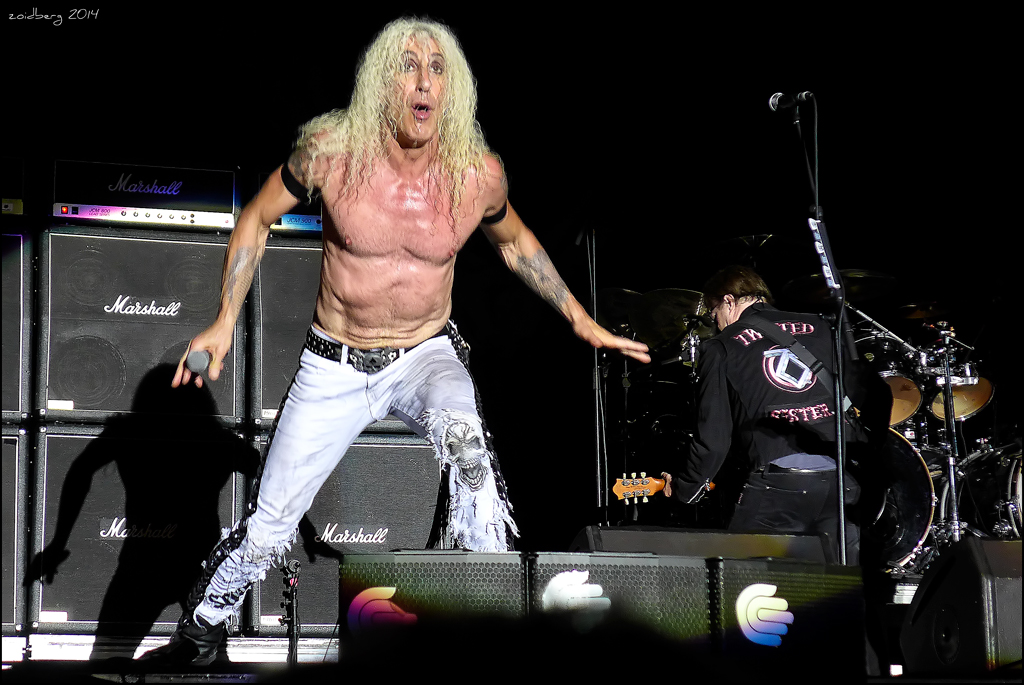In this dynamic stage photo, Dee Snyder, the iconic lead singer from Twisted Sister, commands attention with his wild, long, wavy blonde hair and intense performance energy. Standing shirtless, his broad, tattooed shoulders glisten with sweat under the bright stage lights. Snyder clutches a cordless microphone in his right hand, appearing to scream into it with fervor. His rugged appearance is accentuated by a pair of ripped jeans featuring a distinct smiling skull design on the left knee and a black studded belt with a skull buckle. His outfit is completed by black shoes and black bands around his upper arms. Behind him looms a formidable wall of Marshall amplifier speakers, contributing to the concert's high-octane vibe. To Snyder's right, an electric guitarist, dressed in a black jacket emblazoned with "Twisted Sister" in pink on the back, plays with his back to the audience, positioned in front of the drum set. A microphone stand next to Snyder is adorned with several guitar picks, further hinting at the chaos of the high-energy rock concert. The scene is dark yet dramatically lit, capturing the raw and powerful essence of a classic Twisted Sister performance.